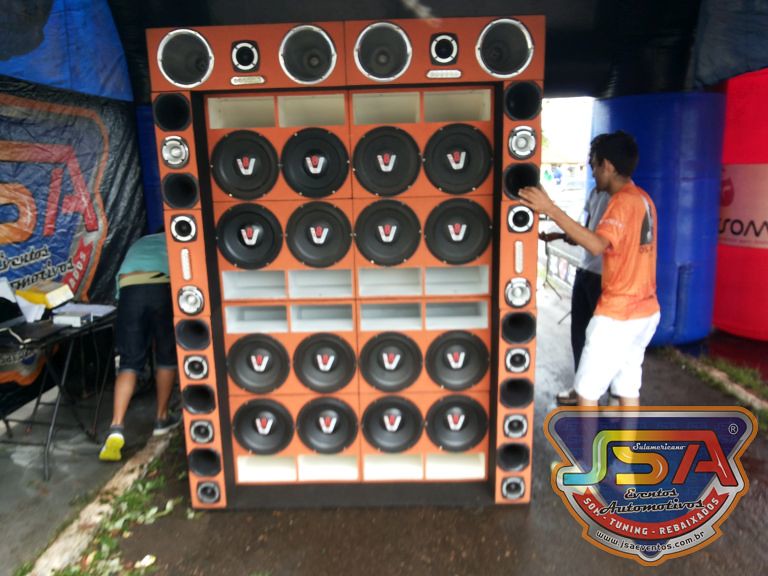The photograph depicts a large display setup in what appears to be a tented area or an oversized garage with a rough concrete floor. The focus is on a cabinet housing an array of variously sized subwoofers and car speakers, arranged in four rows of four. The speakers are predominantly round, black with chrome accents, and orange elements with a distinct V logo. The cabinet also features empty panels designed for head units or controls. The surroundings of the display suggest it's part of an automotive audio event, indicated by a decal in the bottom right corner that reads "Ur Cantos Automotivos" alongside a web address, www.jsaeventos.com.br. The event branding is colorful with yellow, red, and blue, further emphasizing its promotional nature. The walls of the tent seem to be made out of plastic tarp material. The partial presence of three people hints at interaction or inspection of the setup.